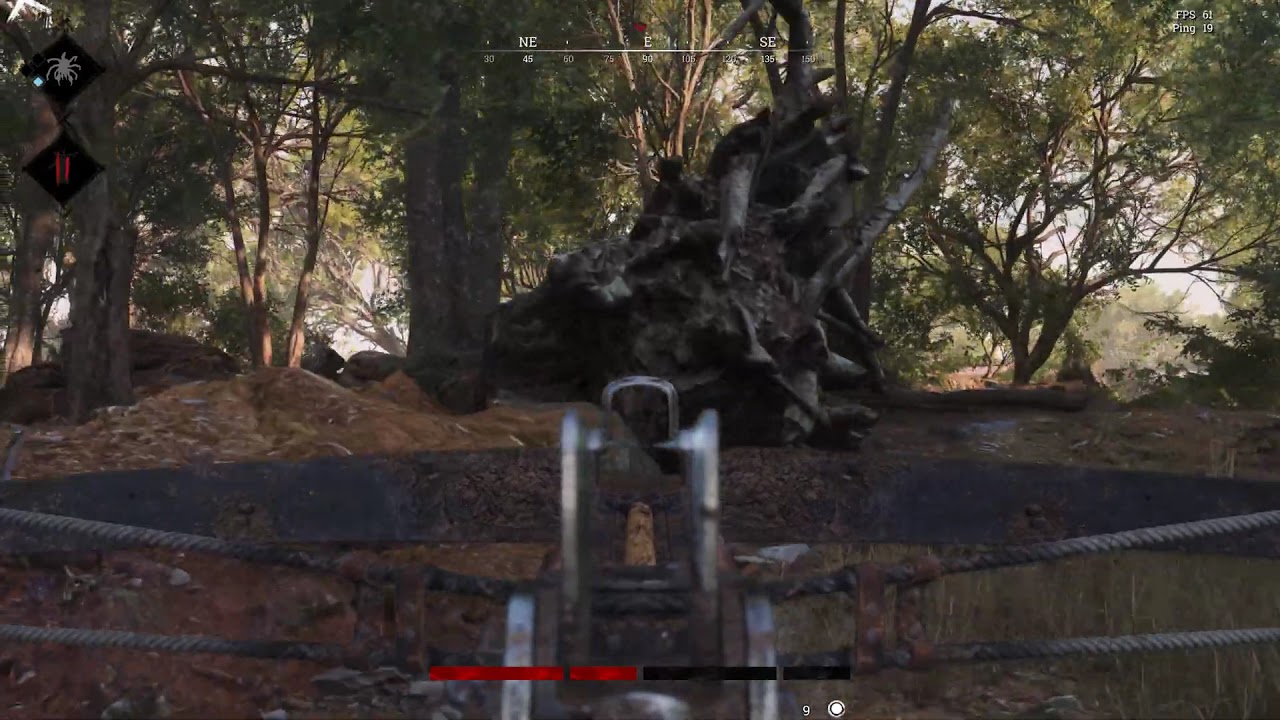The image depicts an extremely realistic screenshot from a first-person shooting video game, presenting the player's perspective through the sights of a weapon that resembles a crossbow or a mounted gun. The weapon is centered in the image, aimed at a dense forest scene filled with trees, fallen timber, and brush. The Heads-Up Display (HUD) features various elements: a scope reticle with distance indicators at the top center, a compass displaying directions like northeast, east, and southeast at the top, and a health bar at the bottom of the screen. To the top left are two black diamond-shaped icons, potentially signifying different gameplay symbols such as a spider. The scene is dominated by earthy tones with greens, browns, and grays, contributing to the overall outdoor ambiance. Despite the detailed environment, there's an absence of any visible people or animals, suggesting the player's current task might be to explore or hunt within the game.